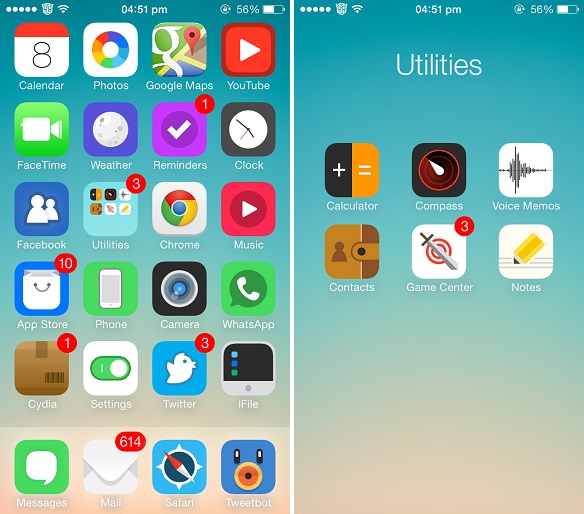This image showcases a cell phone screen with a neatly arranged collection of app icons, commonly referred to as widgets. The widgets are organized in a uniform grid layout, with each row containing four small squares. There are multiple rows of these widgets, creating an orderly presentation.

At the top left corner of the screen, two dots indicate a multi-page layout, followed by an icon resembling a robotic face. To the right of this icon, signal bars provide information about network strength, followed by the current time displayed as 04:51 PM. Further right, a circular arrow surrounding a lock icon signifies screen orientation lock, adjacent to the battery charge indicator showing 56%.

The screen itself is divided into two main sections. The left side is densely populated with apps primarily used for entertainment and social media, including Facebook and YouTube. In contrast, the right side has fewer widgets and is labeled "Utilities." Here, essential tools like the Calculator, Notes, Contacts, and Voice Memos are displayed.

Overall, the image captures a well-organized cell phone interface, balancing essential utilities with leisure and social applications.